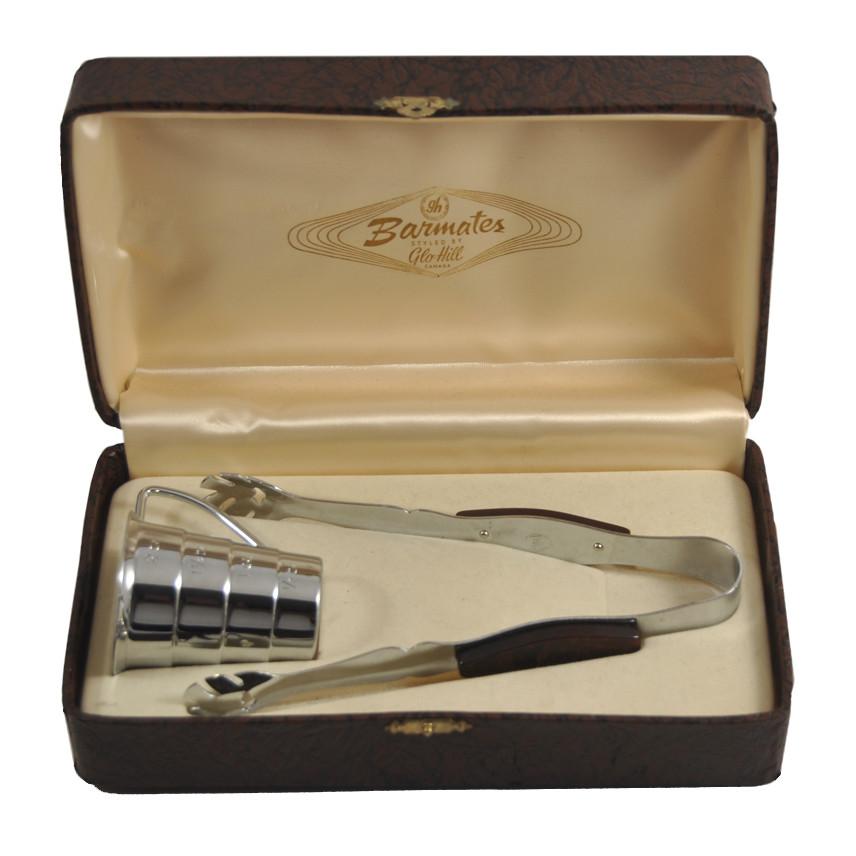The image depicts a rectangular watch-style box with a sophisticated brown leather exterior featuring black detailing reminiscent of leather wrinkles. The box closes with a small gold clasp that rotates over a pin. Inside, the box is lined with a silky, yellowish-cream beige material. The top lid showcases a logo with the text "Bar Mates" surrounded by wavy, oval-ish diamond-style rings, and it also includes the name "Glow Hill" in smaller print. The base of the box contains a stainless steel metal shot crucible with a large handle and a pair of tongs or tweezers. The tweezers have rounded cups with claw-like ends, and their outer edges are adorned with riveted brown grips for enhanced handling.